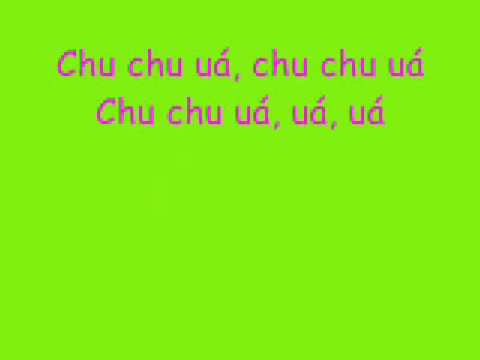The image features a neon lime green background with pixelated hot pink text situated towards the top of the screen. The slightly blurry and low-resolution quality suggests it could be a screen grab from a television or similar electronic display. The text is in a foreign language, reading "Chuchuúa, Chuchuúa, Chuchuúa" on the first line, with repeated "úa, úa, úa" on the second line. Each 'A' in the words has an accent mark above it, adding to the overall electronic and digital feel of the image. There are no other elements present in the image.